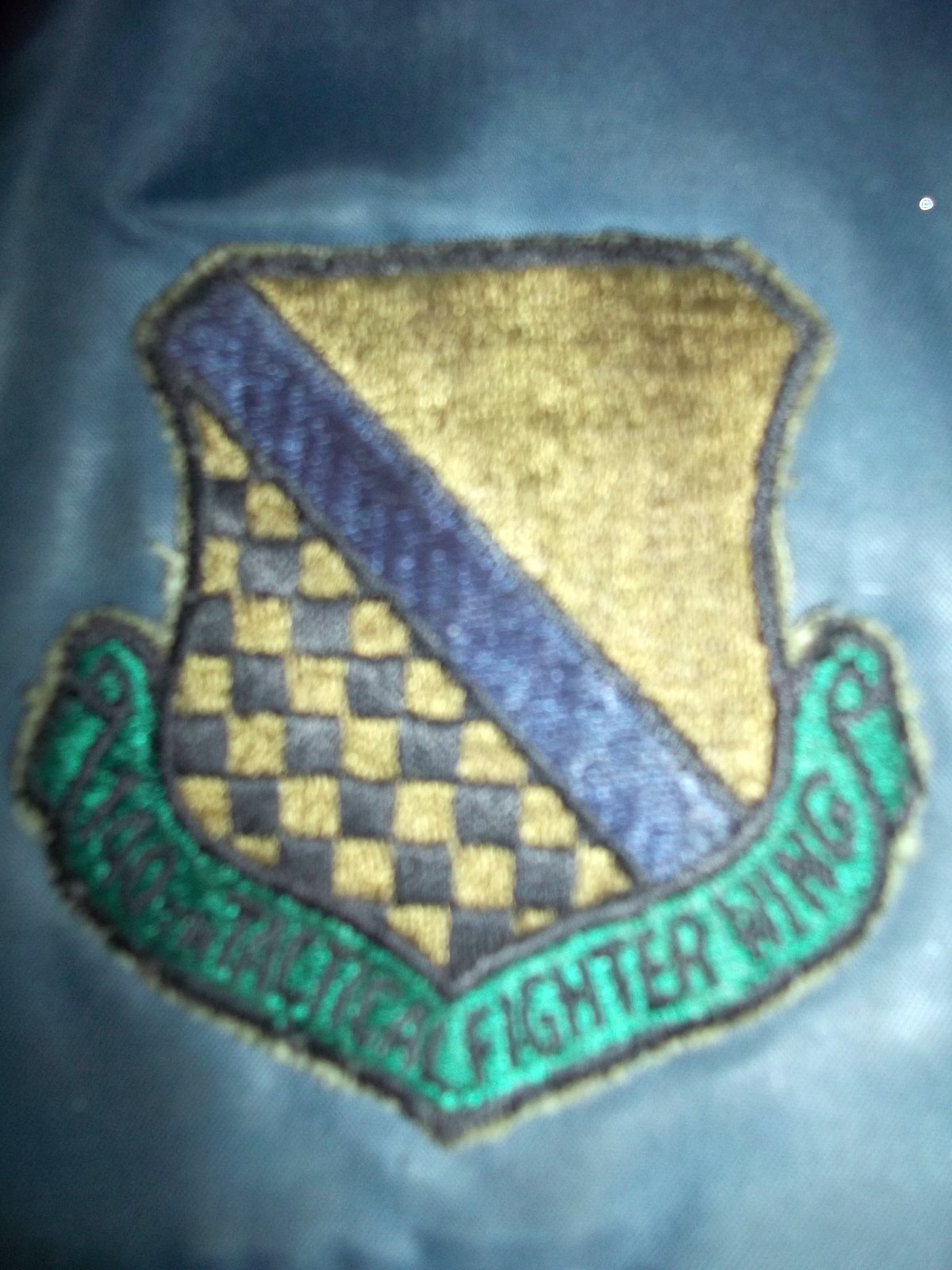The image depicts a close-up of a military patch affixed to the sleeve of a navy blue jacket. The patch features a prominent gold shield with intricate details. A blue diagonal stripe runs from the top left to the lower right of the shield, dividing it into two sections. Below the stripe, there is a checkerboard pattern alternating between yellow and blue squares. The upper part of the shield remains solid gold. Across the center of the patch, a green ribbon with black stitching displays the text "fighter wing" on the right side, while the left side of the text is indistinct. The photograph is full-color but slightly blurry, and appears to have been taken without proper focus. The patch clearly signifies military affiliation, likely indicating the wearer belongs to a fighter wing unit.